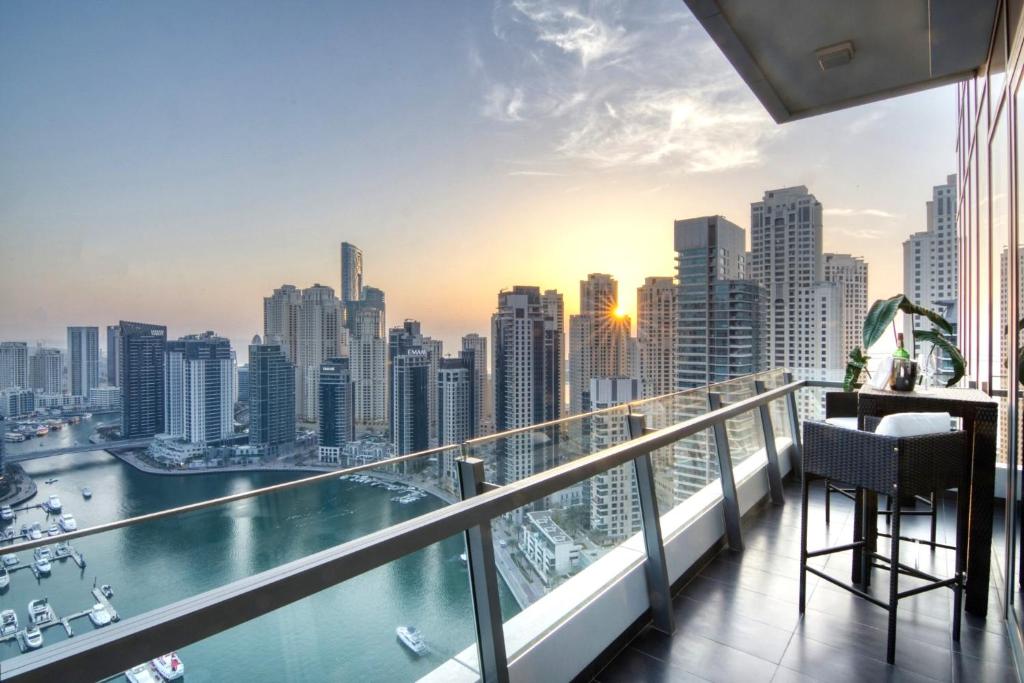This horizontally aligned rectangular picture captures a stunning urban sunset from the vantage point of a high-rise balcony in a city. In the upper portion of the image, a mostly clear blue sky is punctuated by a few feathery white clouds. Dominating the middle of the scene are numerous skyscrapers, varying in shades of gray, dark gray, and white. The sun, a small yellow ball with orange rays, is setting behind one of these buildings, casting a warm glow. Below the skyscrapers, a man-made body of water is visible, reminiscent of Chicago's waterways, dotted with numerous white boats both in motion and docked, particularly in the lower left section. To the left of the water, a bridge is noticeable. The foreground features a balcony with metal bars and glass coverings, a dark gray tiled floor, a wicker basket on a stand with metal legs, and a table with a plant on it, all adding a cozy touch to the urban overlook.